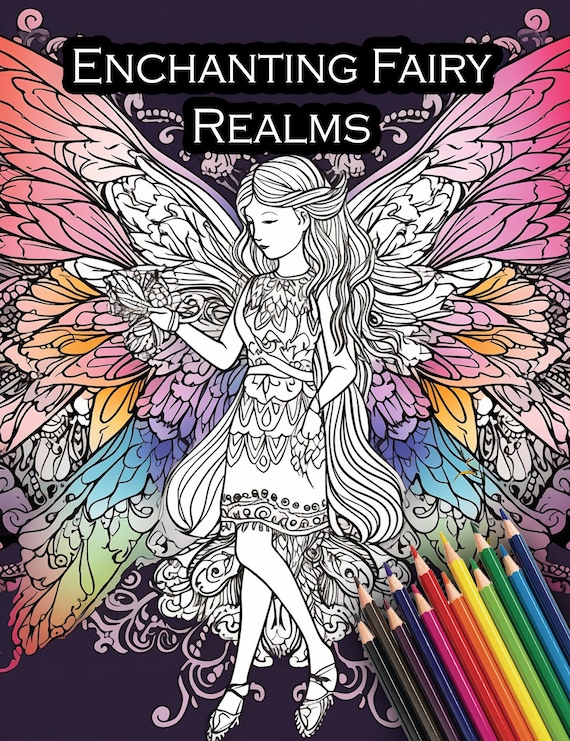The cover of the coloring book titled "Enchanting Fairy Realms" features a beautifully intricate fairy in black and white outline, inviting the colorist to bring her to life. Her partially colored wings exhibit a stunning gradient of hues, including red, orange, pink, light blue, and green, juxtaposing her yet-to-be-colored form. She has long flowing hair and a detailed dress, offering numerous small spaces ideal for an older child or adult to fill with color. The background is a rich dark purple, enhancing the fairy's ethereal presence. At the top, the book’s title is prominently displayed in a black square with white lettering. In the bottom right corner, an array of colored pencils protrudes, showing vibrant tips in colors such as black, brown, violet blue, pink, red, orange, yellow, lime green, green, light blue, and navy blue, ready to be used to complete the fairy's transformation.